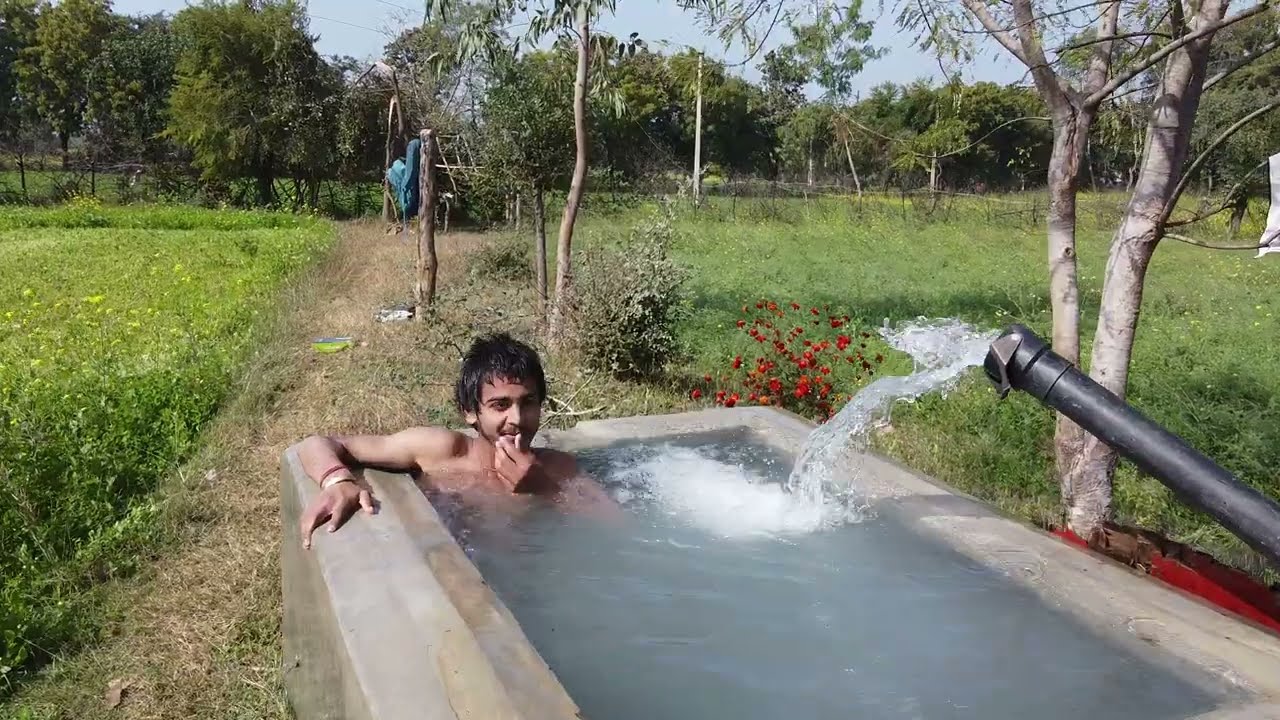The image captures a young man, possibly in his 20s, with medium short black hair and tan skin, sitting shirtless in a rectangular gray vat of water located in an outdoor rural area. The water in the vat rises to his shoulders. The man, who appears to be of South Asian descent, possibly from India, is positioned at the back left-hand side of the vat. His right arm, adorned with bracelets, rests on the edge of the vat, while his left hand scratches his chin, and he seems to be smiling slightly. 

To the right of the vat, a black hose or pipe extends from which water flows into the basin. The surrounding environment features green grass, red wildflowers, and various trees, particularly concentrated in the background. Directly behind the man, there’s a pole with his clothes hanging on it and a well-trodden brown pathway leading towards more vegetation, possibly flowers or crops. Adjacent to the pathway is red machinery and a notable tree that splits into two forks. The scene is under a clear, blue sky, suggesting a peaceful, rural setting where the man might be enjoying a refreshing bath.